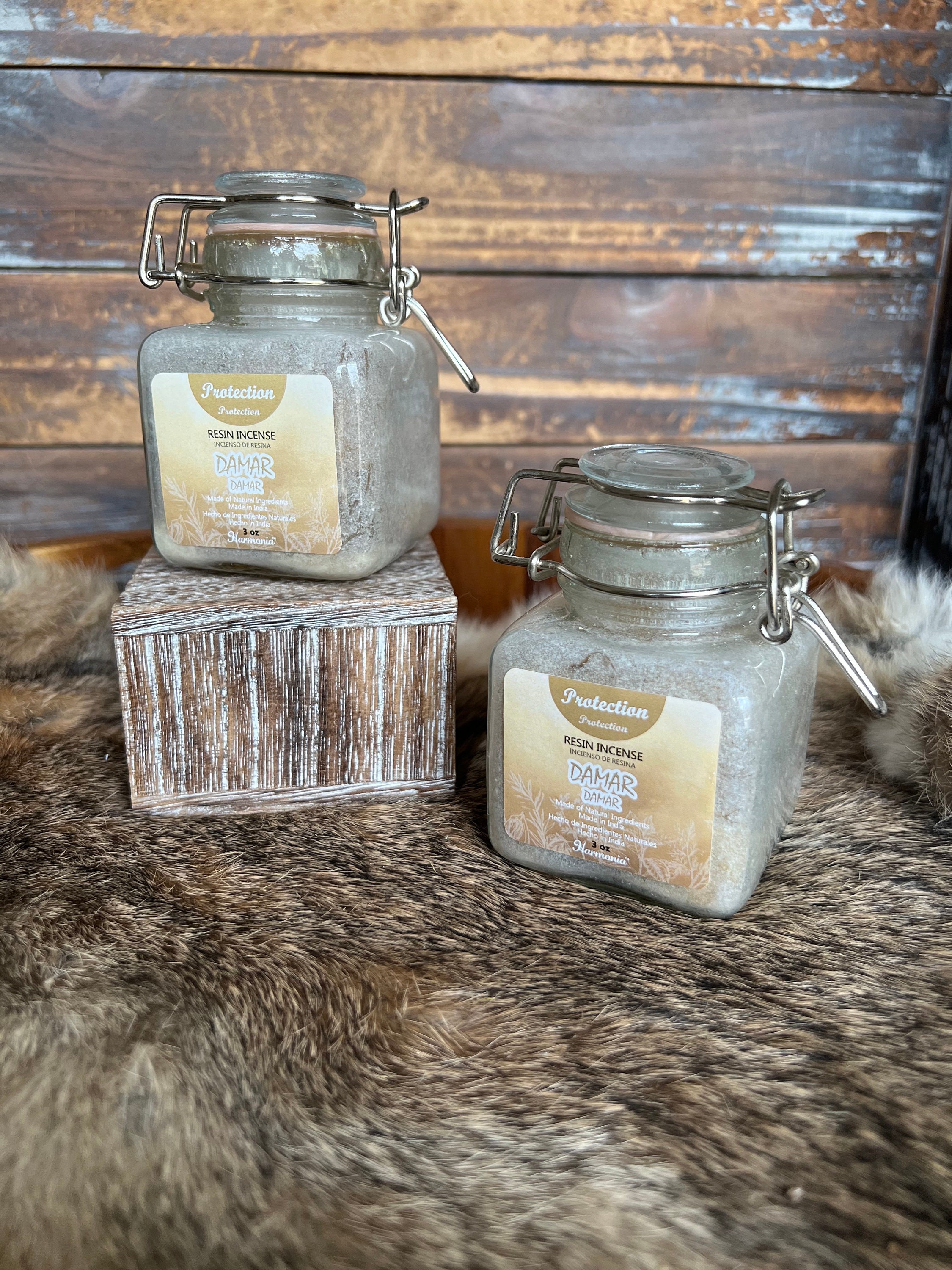This rustic photograph features a scene set against a weathered, old wooden wall, likely from a barn. The backdrop is composed of battered horizontal wooden planks in varying shades of brown. In the foreground, a richly-textured animal skin, possibly a rug, lies sprawled, showcasing tones of brown and light gray. Center stage are two intriguing glass jars that immediately capture attention. These jars are cubic with cylindrical glass tops secured by metal clamps, possibly copper or bronze.

The jar on the left is notably placed on a small, light-colored wooden riser, while the jar on the right sits directly on the animal skin. Each jar contains a powdery substance, possibly sand. Both jars are adorned with almost identical labels—beige with a gradient from a yellowish tan to a darker tan. The labels feature a gold circle at the top with white text that appears to say "protection". Beneath that, in black text, is "resin incense" and "damar damar". Despite the clarity of the photograph, the fine print remains difficult to discern. 

Adding to the scene's charm are small yellow stars, possibly plastic, scattered subtly around the jars, further enhancing the display's aesthetic appeal. This carefully arranged composition, rich in texture and detail, begs for a closer inspection and seems to tell a story that remains just out of reach.